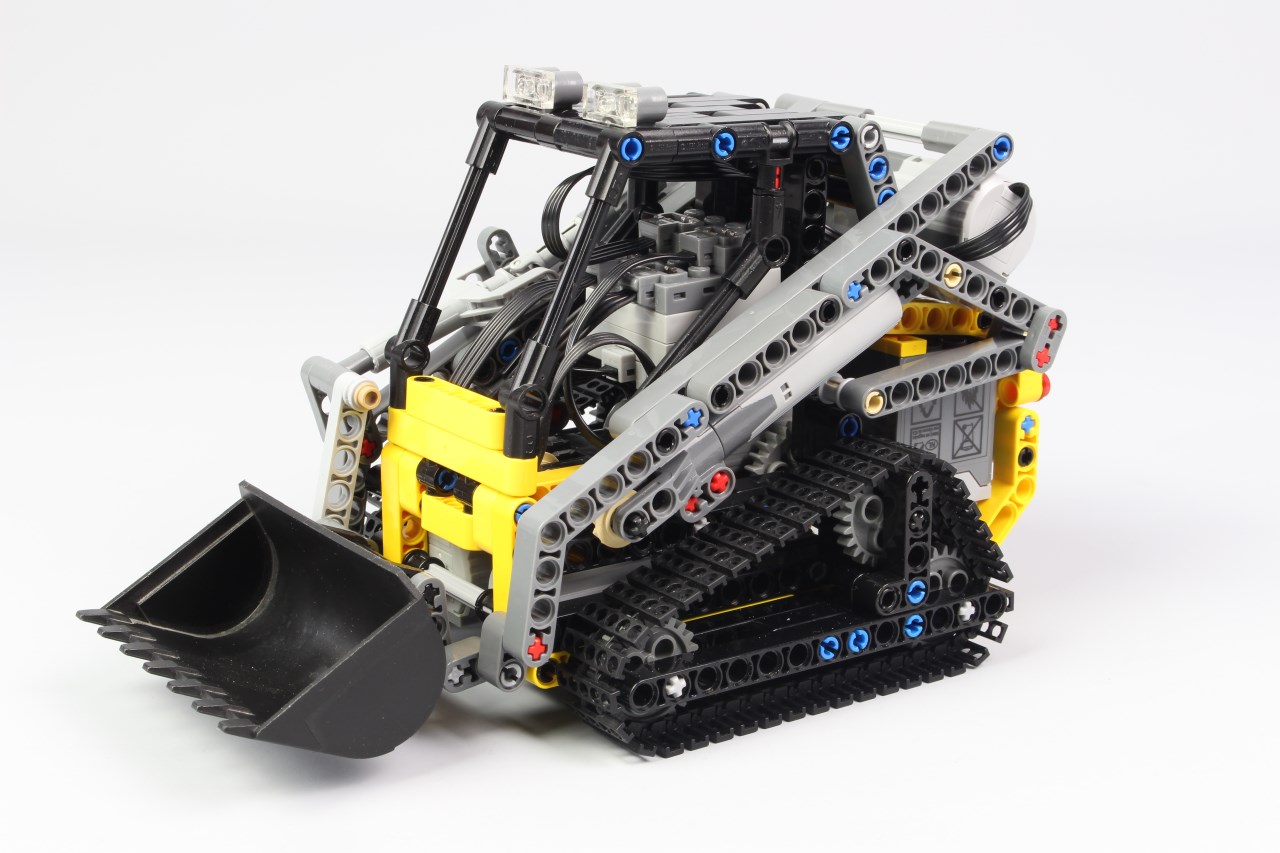The image showcases a detailed toy bulldozer constructed from Lego bricks. The vehicle, which appears highly intricate, features a yellow base and a black wheel track on the bottom, indicative of a bulldozer or digging machine. The majority of the body is composed of yellow, gray, and black plastic pieces, creating a realistic and functional appearance. The cabin of the bulldozer is encased in black plastic with blue accents that resemble screws, ensuring the structural integrity of the model. The front of the vehicle includes a black scooper, equipped with ridges and prongs designed to simulate dirt-moving capabilities. Two headlights are mounted on the top, presumably to illuminate the path ahead. The image is set against a white background, highlighting the impressive craftsmanship of the Lego bulldozer.